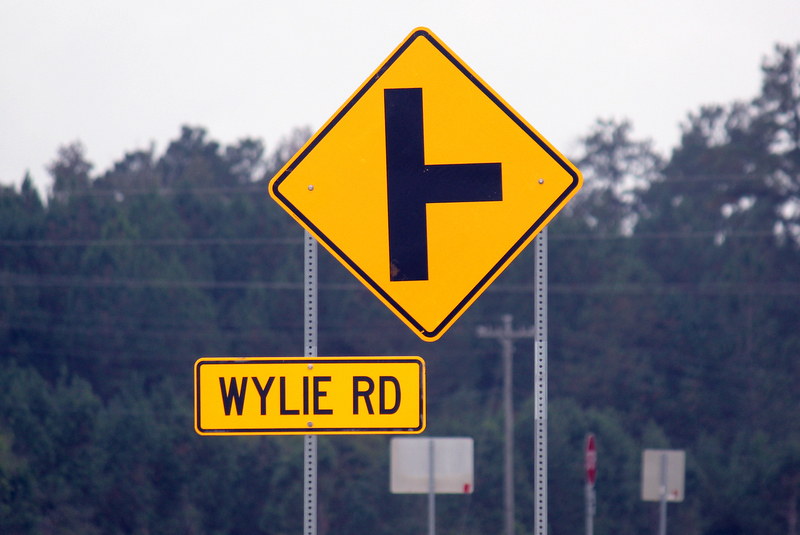The image features a prominent yellow traffic sign indicating an intersection, specifically a T-intersection where the road tees off to the right. The sign is diamond-shaped with a bold black outline. Below this primary sign is a rectangular yellow sign bordered in black, displaying the text "Wiley Road" in capital letters. Both signs are mounted atop two metal posts anchored in the ground. To the right of this setup, in the background, is a square road sign with additional signage in its vicinity, including a horizontally oriented stop sign. The scene is further set against a backdrop of power lines and evergreen trees under an overcast, light gray sky.